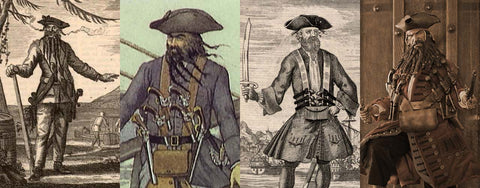The image consists of four small rectangular illustrations of Blackbeard the pirate, arranged in a row. The first illustration, in black and white or a cream tone, depicts Blackbeard standing outdoors with his hands extended, holding a cane or wooden stick. The second image, with a green background, provides a close-up of Blackbeard on a ship, wearing a blue coat, pirate's hat, long braided beard, and a brown harness across his chest adorned with several pistols. The third illustration, also black and white, features Blackbeard in a tunic-like outfit, holding a sword upright in his right hand. The final image on the far right, rendered in a brownish tint, shows Blackbeard seated, gazing over his left shoulder, with a flowing beard and a brown pirate hat. Collectively, these detailed renderings provide a multifaceted visual portrayal of the infamous pirate.